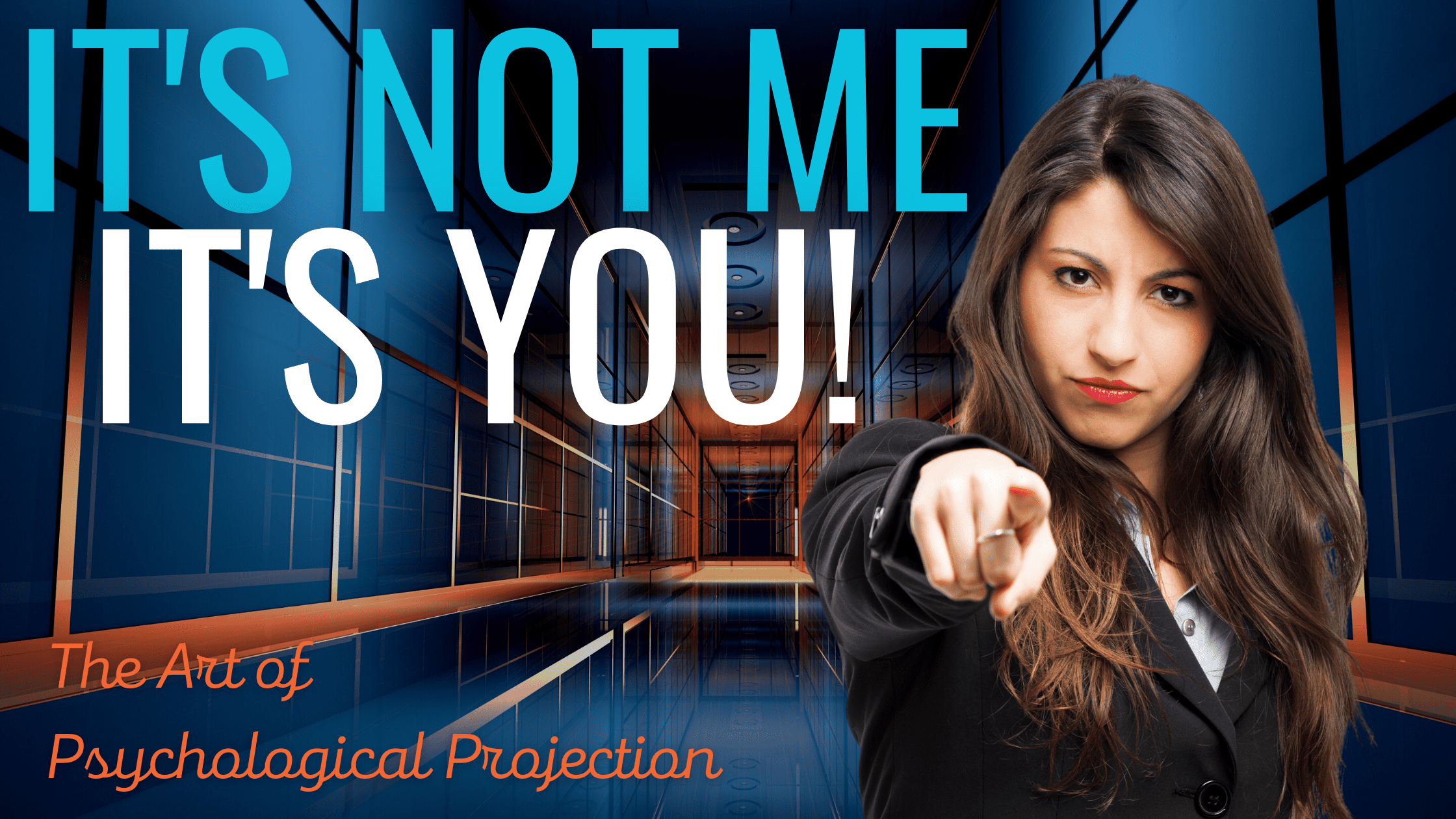The image appears to be an advertisement or promotional material, potentially for a course or lecture on psychological projection. Dominating the upper left portion of the image, the phrase "IT'S NOT ME, IT'S YOU!" is boldly written, with "IT'S NOT ME" in large turquoise letters and "IT'S YOU!" in large white letters followed by an exclamation mark. Below this, in script-like orange or red lettering, the text reads "The art of psychological projection."

To the right of the text stands a young Latina woman with long, dark hair and red lipstick. She is dressed in business attire, possibly a double-breasted coat, and has a stern look on her face as she points directly at the viewer. The image gives prominence to her serious expression and direct gesture. On her middle finger, there appears to be a gold ring.

The background of the image consists of a CGI-rendered hallway that features geometric shapes and reflective blue panels interspersed with brownish-orange beams or connectors. The reflective floor adds depth to the setting, emphasizing the futuristic or abstract design of the corridor. Overall, the woman's commanding presence and the striking text combine to create a compelling and intense visual message.